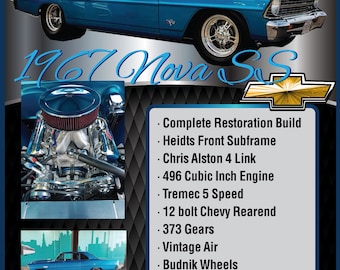This image features an advertisement for a meticulously restored 1967 Chevrolet Nova SS. Dominating the upper portion, the vibrant blue car is partially visible, showcasing its front end with a silver fender, illuminated headlights, and two polished wheels. Below, "1967 Nova SS" is prominently displayed in elegant blue lettering, accompanied by the iconic Chevrolet emblem in gleaming gold, resembling a cross. Enclosed within a light gray rectangle, a comprehensive bullet list details the car's impressive features: a complete restoration build, Heights front subframe, Chris Alston 4-Link, 496 cubic inch engine, Tremec 5-speed transmission, 12-bolt Chevrolet rear-end, 3.73 gears, Vintage Air conditioning system, and Budnick wheels. Adjacent to these specifications, to the left, are detailed photos including a close-up of the car and its robust engine, illustrating the superior craftsmanship of this antique turquoise-colored vehicle.